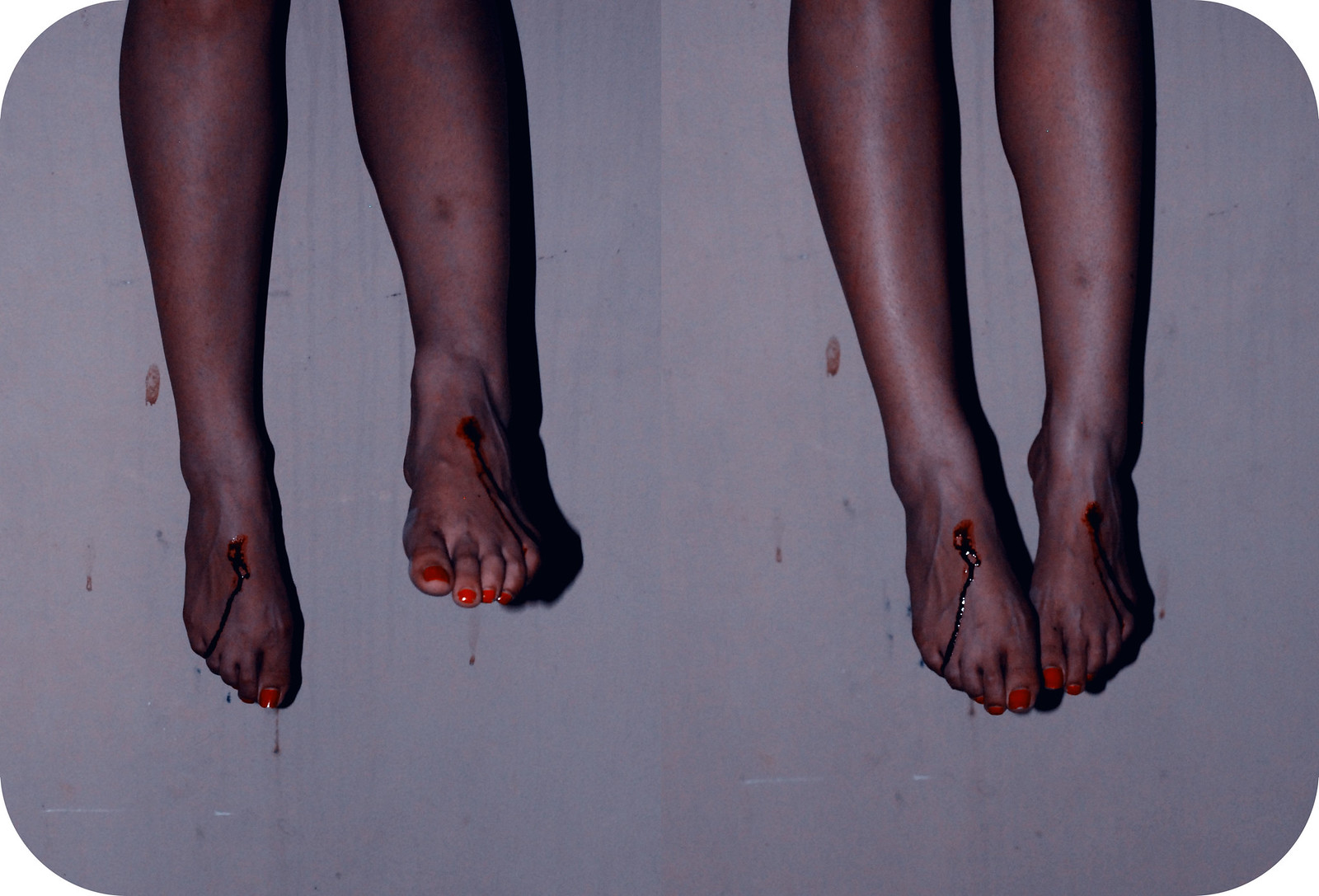The image depicts a chilling scene featuring two pairs of women's feet and the lower halves of their legs, prominently filling the entire frame. The photograph itself has curved edges. Captured from the knees down, both sets of legs are positioned in an unsettling manner reminiscent of a crucifixion, suggesting they are hanging against a white wall. Both women have large, traumatic wounds on the tops of their feet with blood visibly running down to their toes, splattering and dripping onto the wall below. Nails, possibly used to inflict the wounds, are either obscured or have been removed, enhancing the gruesome effect. Despite the gruesome injuries, both pairs of feet share a common detail: their toenails are meticulously painted in a glossy, bright red nail polish.